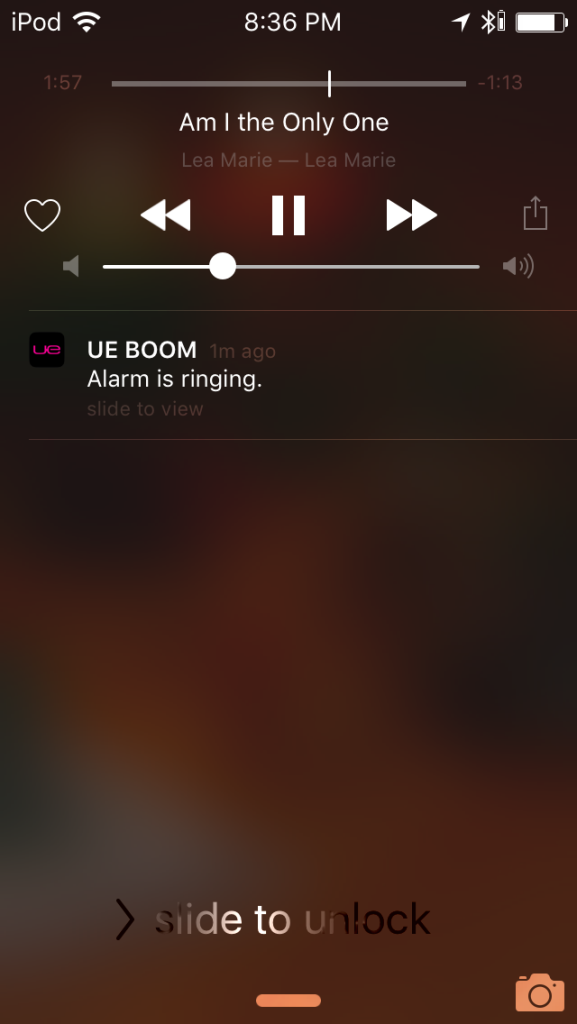The image captures a blurred printout of an iPod screen. In the top left corner, the word "iPod" is prominently displayed next to a signal indicator. Directly below the signal indicator, the time reads "1:57". Adjacent to the word "iPod" on the right side, another time is displayed as "8:36 PM", followed further to the right by various icons including a battery life indicator. The screen indicates that the song "Am I the Only One" by Lea Marie is currently playing. A heart-shaped icon and a volume indicator are also visible. Just below, text reads "UE Boom alarm is ringing" followed by "Slide to view, one minute ago". At the bottom of the screen, the instructions "Slide to unlock" are clearly visible. Additionally, next to the "UE Boom alarm is ringing" text on the left, there is a hot pink icon set against a dark black background.